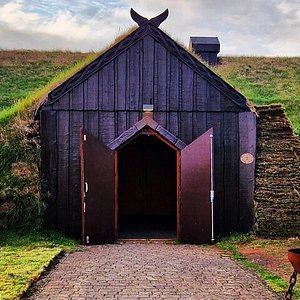This outdoor photograph captures a barn built into the side of a low hill, viewed from the ground level. The sky above is predominantly covered in grey and white clouds, with slivers of light blue peeking through. The barn, constructed of vertically slatted brown wood, is front and center. Its dark blue or burgundy doors are open wide, revealing an interior enshrouded in darkness. Notably, the doors feature a pitched opening at the top and are bordered in a darker hue of blue or purple, crisscrossed by wooden trim. At the peak of the barn's roof, a wooden carving of an eagle with wings spread out adds a rustic charm. Vegetation such as grass and possibly hay grows on the right side of the roof, enhancing its integration with the natural hill. In front of the barn, a cobblestone walkway extends to the bottom of the image, flanked by lush green grass on the left and a dirt path on the right. The surrounding environment is alive with patches of grass and occasional rocky outcrops, embodying a serene countryside landscape.